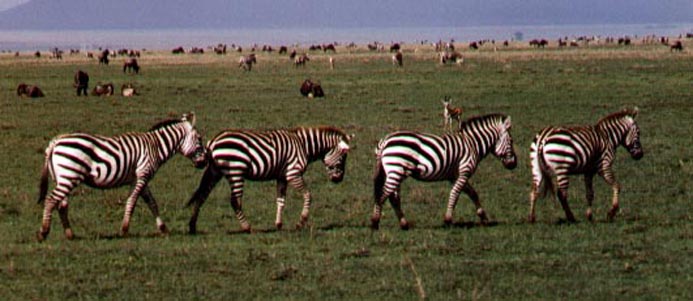In this outdoor landscape photograph, taken in what appears to be a grassy field or meadow, a captivating scene unfolds under a partly cloudy sky. In the foreground, four zebras with striking black and white stripes march in a straight, orderly line from the left to the right side of the picture. Their short, matching black and white striped manes add to their distinctive appearance. The grass where they tread is lush and green, though farther in the background, it transitions to a drier, more yellow hue, suggesting a change in terrain near the distant lake or ocean that is just barely visible. Scattered further back in the image are various other animals, including some antelopes with babies, and what appears to be buffalo or bison resting on the ground. This diverse assembly of wildlife collectively forms an intricate tableau, creating a rich and dynamic portrait of a verdant habitat.